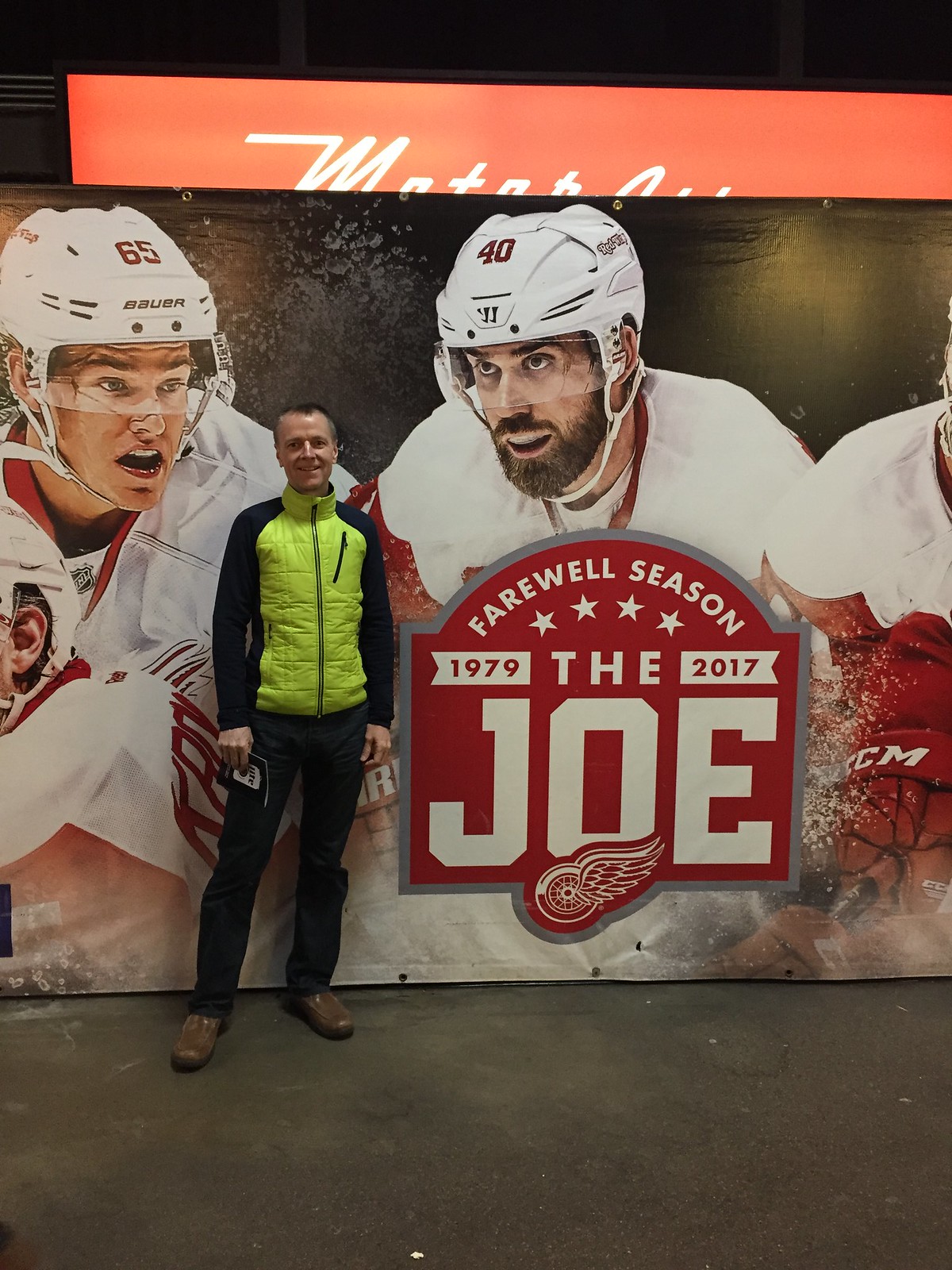In this portrait photograph, a man in his late 50s stands in front of a detailed banner. He wears a vibrant lime green zip-up jacket with black sleeves, black pants, and brown shoes. His short, brownish-gray hair suggests his mature age. The banner behind him, prominently colored in red, gray, and white, displays the text "Farewell Season 1979-2017 The Joe," commemorating the farewell season of Joe Louis Arena. The backdrop also features images of hockey players in white jerseys and helmets with red accents, identified by their numbers—65 on the left, 40 in the middle, and another player to the right. The floor below is pavement-like, indicating the photo was likely taken at the stadium during a hockey game.